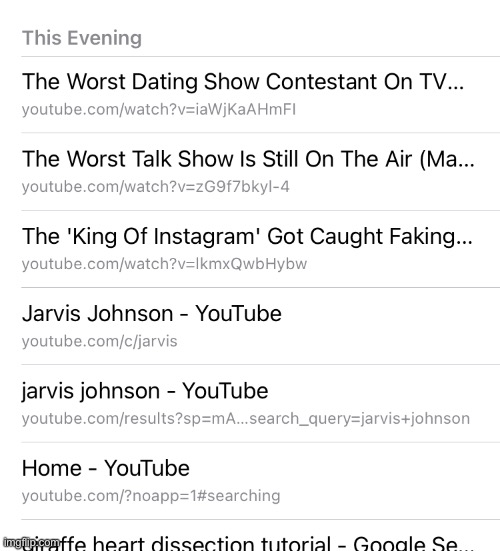On the webpage, a series of captions are displayed on a white background with gray text. At the top, it reads "This evening" followed by a thin gray line. Below the line, various statements are sequentially listed in gray text:

1. "The worst dating show contestant on TV... you can watch it on YouTube."
2. "The worst talk show is still on the air (MA)... that's also on YouTube."
3. "The 'King of Instagram' got caught faking... again, it's on YouTube."
4. "Jarvis Johnson - YouTube on youtube.com"
5. "Jarvis Johnson - YouTube on youtube.com" (This appears twice, once with 'Jarvis Johnson' capitalized and once not capitalized).
 
Under these, additional text is displayed:

- "Home - YouTube youtube.com"
- "Giraffe heart dissection tutorial Google se"

Additionally, a white stamp on the page reads "IMGFIPI.com".

This detailed yet structured overview captures all visible elements, providing clarity on the webpage's content and layout.